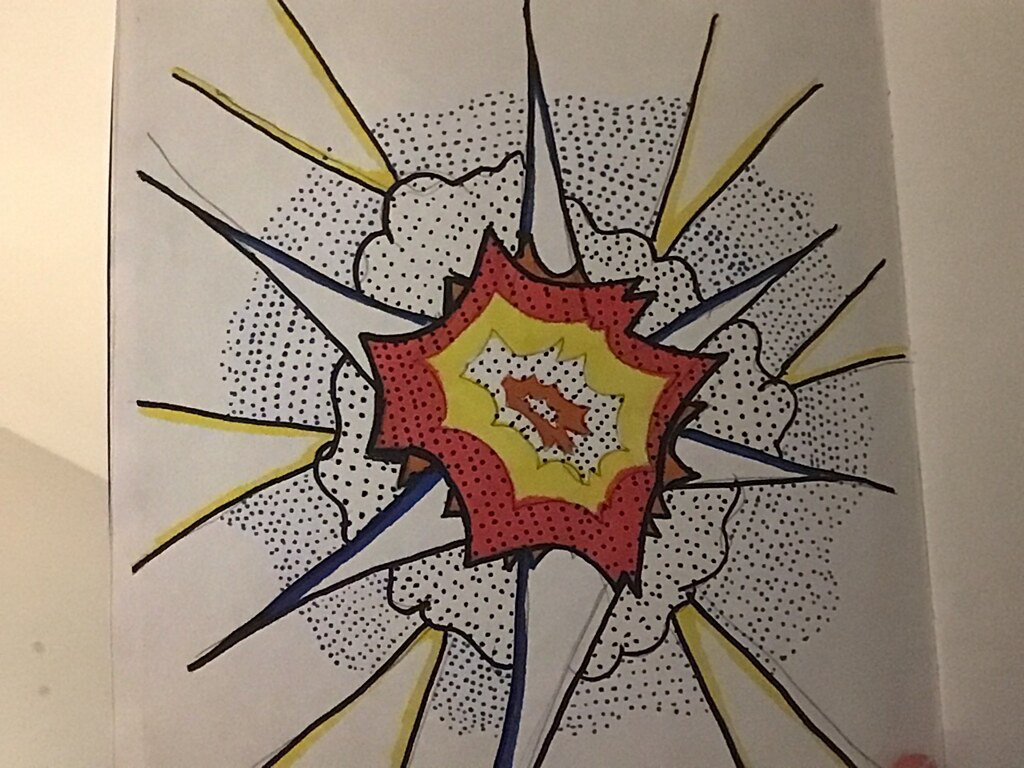The photograph captures a vibrant graphic design illustration, potentially serving as a logo or an abstract artwork. Central to the composition is a bold, comic book-style explosion cloud with dynamic rays emanating outward. A prominently featured letter "A" sits at the heart of the explosion, encircled by a striking combination of yellow and red fire effects, adding a sense of energy and intensity to the design. The illustration is rendered on plain white paper, placed on what appears to be a white surface, likely a desk or table. Ambient and directed light, possibly from a desk lamp, cast shadows and highlights across the scene, enhancing the visual appeal. Additionally, the bottom of the image reveals a partial view of a person's finger pressing against the paper, hinting at the artist's interaction with their work in a personal drawing space, presumably within their home.